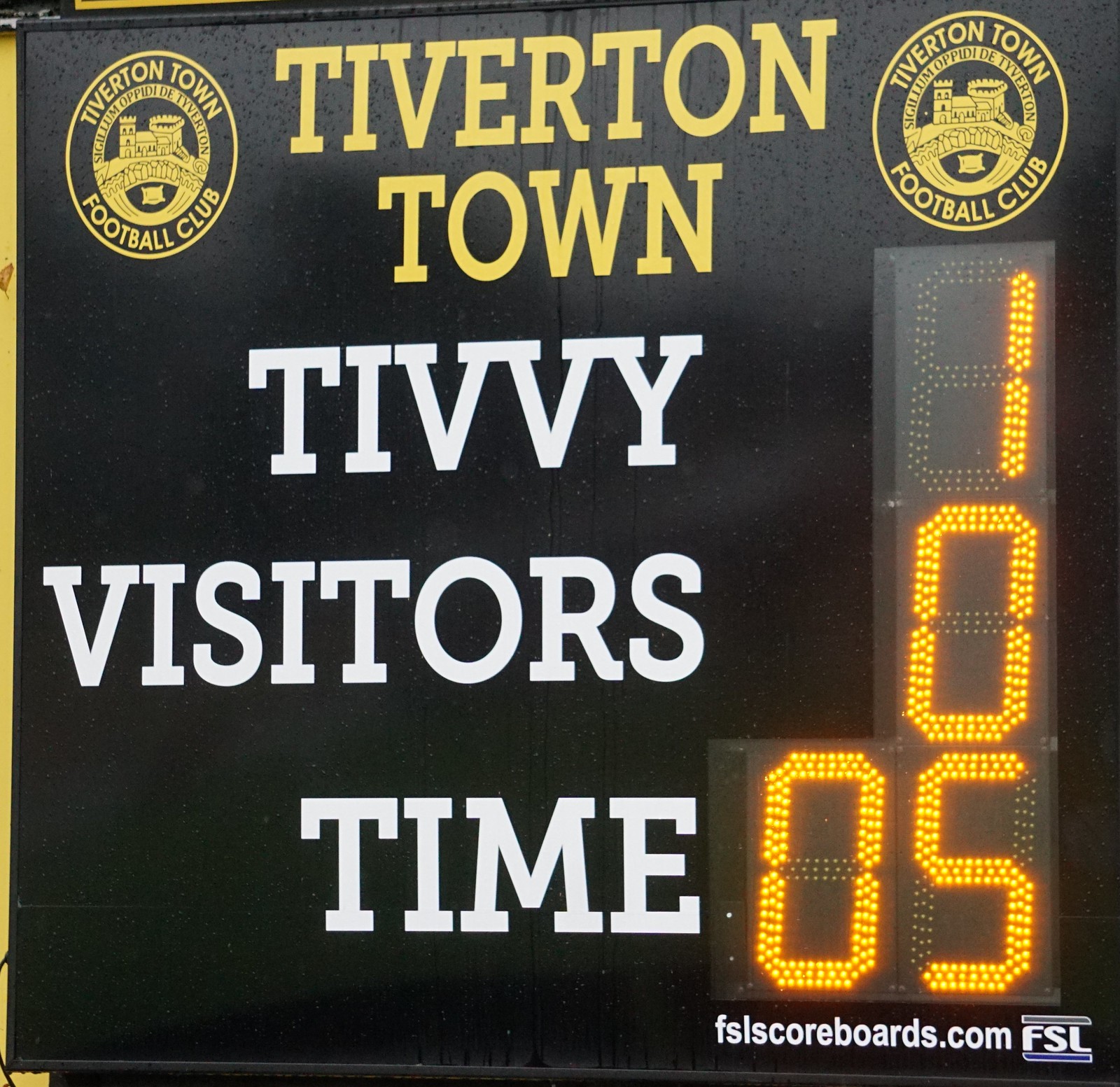This detailed image captures a scoreboard prominently displayed against a black backdrop. The scoreboard is for Tiverton Town Football Club, featuring minimal but striking colors—gold, white, and an orange-yellow. At the top center, the text "Tiverton Town" is showcased in a bold gold color. Flanking this text on both the left and right are the club’s logos, each resembling a seal containing Latin text, "Siglum opidi de Tiverton," alongside a depiction of a castle.

The game details are clearly presented in the middle section: the home team labeled "Tivvy" in white text has scored 1, displayed in bright orange digital numbers. Directly below, "Visitors" are shown to have a score of 0, also in white text. The current time of the game is marked as "05" in white. Underneath these details, the scoreboard features the website FSLScoreboards.com and the initials "FSL" in a small logo form, adding a subtle branding element.

The simplicity of the design, with its limited text and colors, suggests it was likely captured by a bystander attending the game, emphasizing the essential game statistics with clarity and focus.